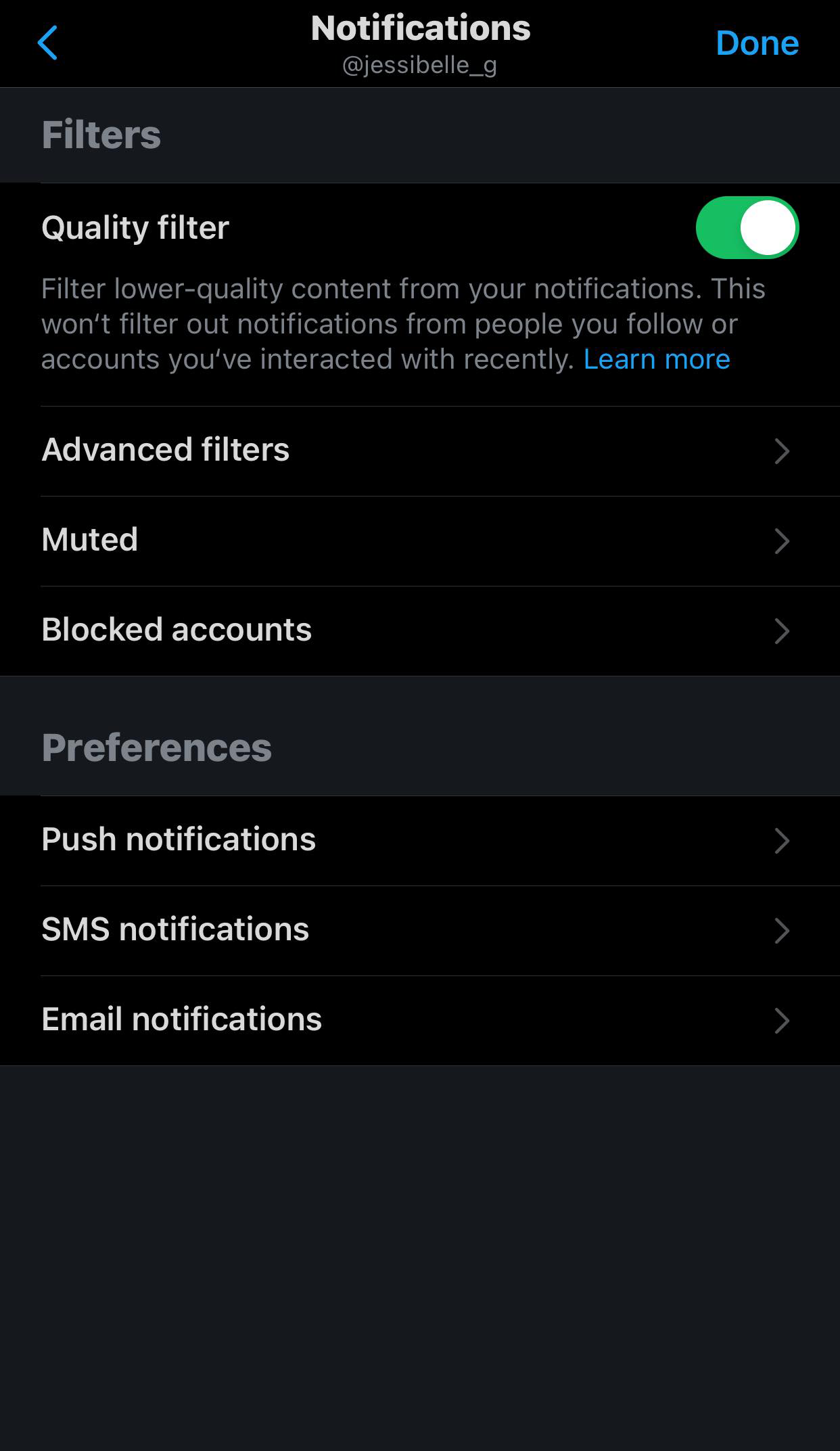The image appears to be a screenshot from a mobile device, likely a tablet or smartphone, displaying a notifications settings page from an application. The screen features the username "@jessabelle_g" prominently at the top, with a blue arrow pointing to the left, indicating a back button. To the right, there is a highlighted blue "DONE" button.

Below this top section, the screen is divided into various headings and filter options:

1. **Quality Filter**: This section has a blue toggle switch indicating that the quality filter is turned on. The accompanying description explains that this filter will remove lower quality content from the user’s notifications, without affecting notifications from followed accounts or recently interacted accounts. A blue "Learn More" button is present for additional information.

2. **Advanced Filters**: Under this heading, there are options for managing muted and blocked accounts.

3. **Preferences**: This section provides settings for push notifications, SMS notifications, and email notifications.

The screen is devoid of any background or surroundings, focusing entirely on the application’s settings.